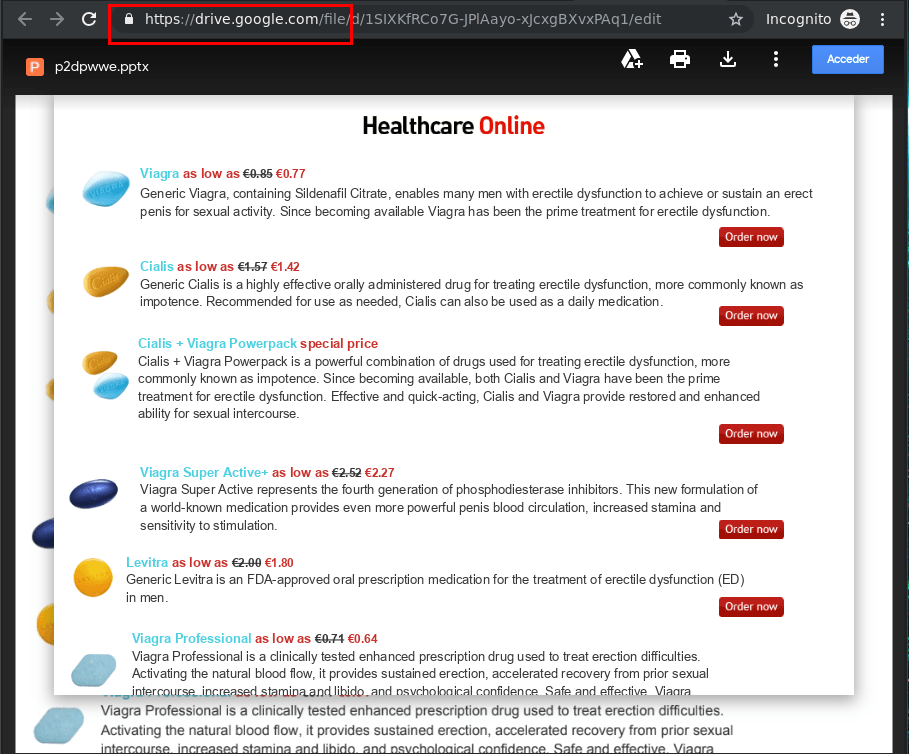The image consists of a black background overlaid with various elements. At the top, there is a prominent white square. Within the black portion at the top, there's a red-outlined button featuring the address "drivegoogle.com." In the top-right corner, a blue rectangular button is labeled "Assetto."

Beneath these elements, the words "Healthcare Online" are prominently displayed, with "Healthcare" in bold black letters and "Online" in bold red letters. The content includes a list of medications: "Viagra," "Silas," "Silas Plus Viagra Power Pack," "Viagra Super Active," "Levitra," and "Viagra Professional."

Each medication is accompanied by descriptive paragraphs specifying their uses. Beside these descriptions, images of the pills are displayed in the following color patterns: blue, gold, gold and blue, darker blue, and gold and lighter blue.

Additionally, each paragraph is paired with a red button containing the text "Order Now" in white.